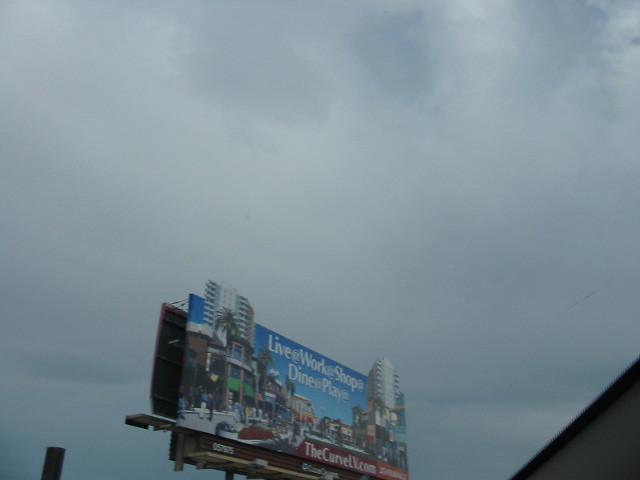This detailed photograph captures a striking view of a cloudy light blue sky filling most of the frame, punctuated by prominent, fluffy clouds. In the bottom right corner of the image, a dark-colored building makes a partial appearance, cut off by the edge of the frame. Dominating the lower third of the photograph is a billboard, slightly off-center to the left. The top middle section of the billboard features the text: “Live at, Work at, Shop at, Dine at, Play at,” inviting viewers to embrace a vibrant lifestyle. Below this enticing message, the words “thecurvelv.com” are visible, followed by additional text that remains unreadable from this vantage point. The billboard itself showcases a lively tropical street scene complete with towering colorful buildings, some reaching skyscraper heights. Palm trees line the street, providing a picturesque backdrop for the multitude of people leisurely strolling by various shops and establishments. In contrast to the cloudy sky of the photograph, the sky within the billboard glows a brilliant blue, enhancing the dynamic and inviting atmosphere of the scene depicted.